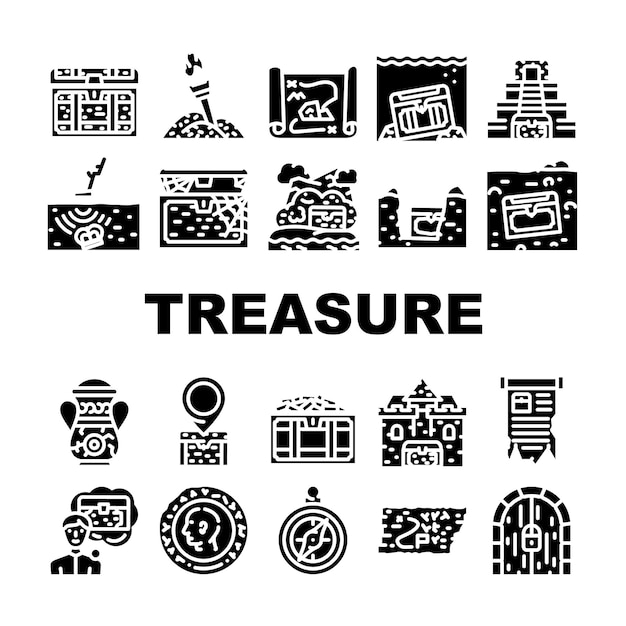This black-and-white image features a collection of 20 small clipart icons related to treasure, arranged in four rows of five against a solid white background. The upper and lower sections each contain two rows of detailed black icons, uniformly spaced apart. These icons frame a central gap that showcases the bold, uppercase word "TREASURE" in large, black block letters.

In the upper left corner, an outlined treasure chest with its lid partially open catches the eye, while to its right, a flaming torch adds an adventurous flair. Other notable icons in the top rows include a treasure map, symbols, and a stairway ascending to a door in the upper right corner. The lower left begins with an outline of a person with a thought bubble, positioned beneath a vase. Nearby, there's a coin with an engraved head, a clock, and an arched doorway in the lower right corner.

Additional icons scattered throughout the image include various treasure chests, some hidden behind cracks in walls, some underwater, on hills or mountains, and even buried underground. Treasures aren't the only focus; there's also a step pyramid, a castle, symbols suggesting alien design, a compass, and more, all contributing to the theme of hidden riches and exploration.